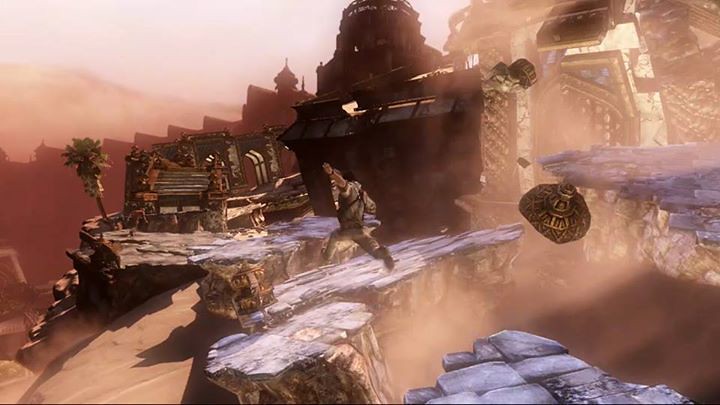In this vividly imagined scene, possibly inspired by a video game, a lone character is seen sprinting across a rugged cliffside platform that is part of a vast mountainous landscape. Dominating the foreground is a peculiar building featuring a large, open, black garage; its dark interior hints at hidden, perhaps ominous contents. Flanking this structure on the left are several rugged, brown vehicles equipped with mountain-climbing gear, ready to conquer the steep terrain. Leaning slightly to the left, a single palm tree with vibrant green fronds adds a touch of tropical contrast to the otherwise harsh environment.

Further enriching the scenery is an unusual sight: a gold bag hangs from one of the clouds, gently swaying in the atmospheric currents. In the background, a cluster of additional houses nestles against the mountainside, creating a sense of a hidden, thriving community amidst the wilderness. Beyond these dwellings, a golden structure—perhaps another segment of a larger building—glistens on a distant peak, hinting at secrets and treasures yet to be uncovered. This imaginative tableau captures a world where adventure and mystery seamlessly blend into the dramatic natural surroundings.